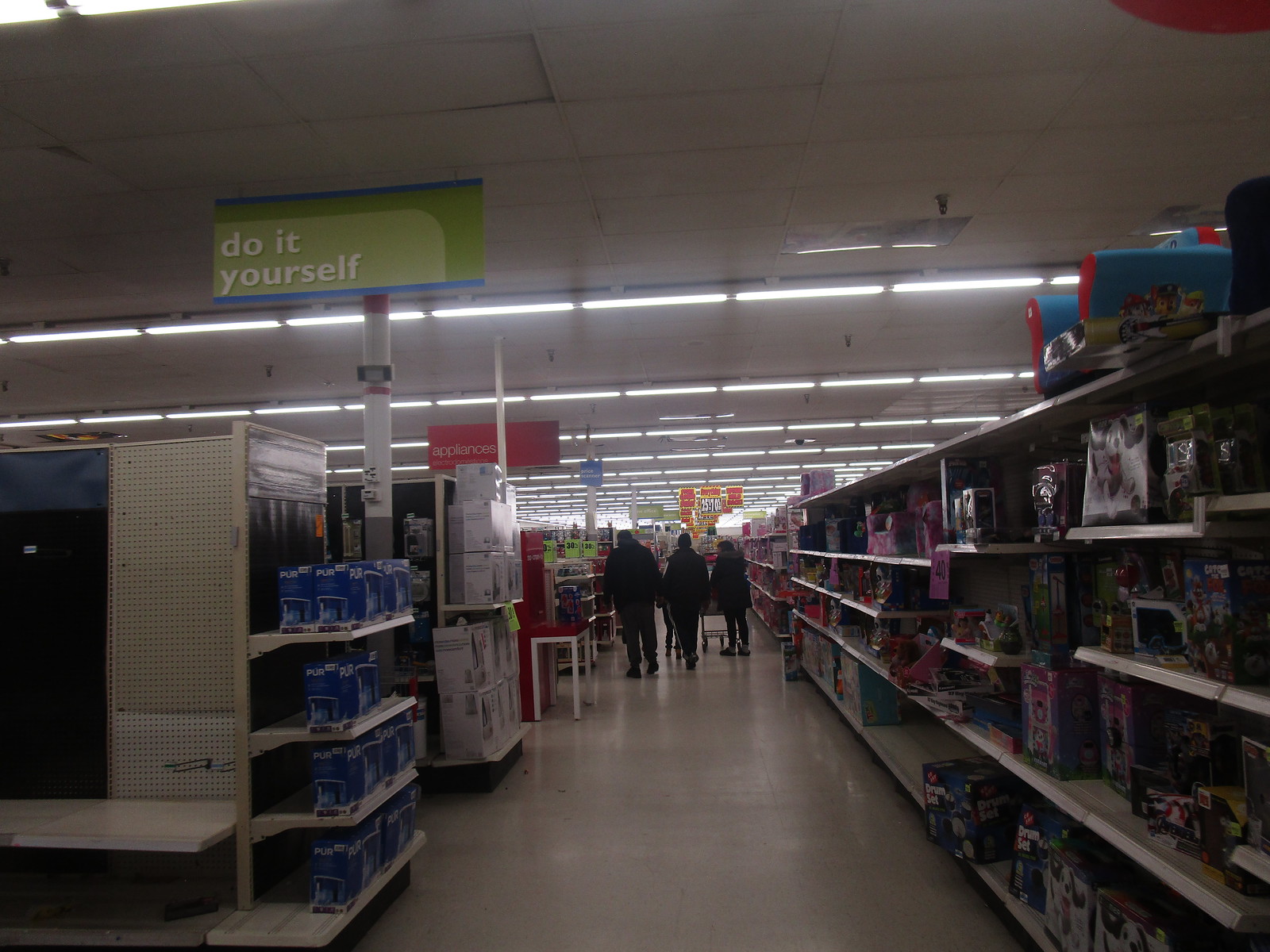The photo depicts a spacious aisle inside a department store, reminiscent of a Walmart or Target, illuminated by rows of horizontally aligned fluorescent light bulbs that stretch as far as the eye can see, creating a dimly lit atmosphere. The ceiling features white drop tiles and is adorned with a green rectangular banner that says "Do It Yourself" and a red rectangular banner further down that reads "Appliances." The aisle has tan linoleum flooring, flanked by typical tan metal store shelving loaded with various merchandise. In the foreground, three people, appearing as shadowy figures due to the lighting, walk down the aisle away from the camera. One person on the far right side is pushing a shopping cart, and among the group is a child between two adults. The scene captures the essence of a bustling department store aisle, teeming with products and highlighted by clear signage indicating different sections.